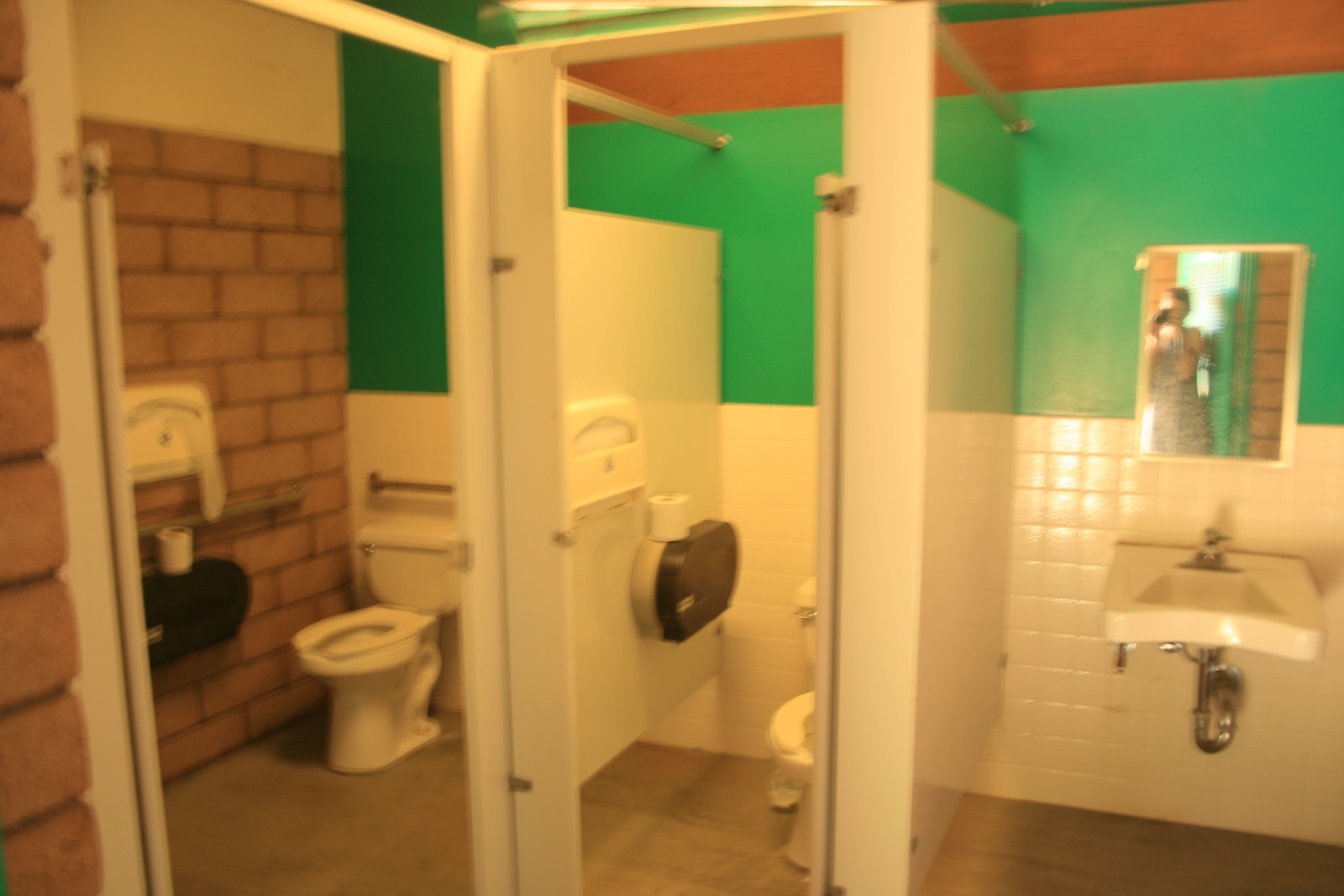The photo depicts an eclectic bathroom with unique color schemes. On the left side, there's a yellow brick wall, likely drawn or fake, and in front, the wall features a combination of white tiles on the lower half and a lime green painted section above, topped with a wood-toned section. The floor is entirely tiled. To the left, there's a larger handicapped-accessible stall with an angled door, housing a toilet, a toilet paper dispenser, and a toilet seat cover holder. Next to it, there is a narrower stall with similar amenities. On the right side, a white sink with silver piping sits beneath a mirror, which reflects the photographer and shows a door open behind them, indicating daytime with sunlight casting shadows. The image itself appears fuzzy and grainy, contributing to its overall character.